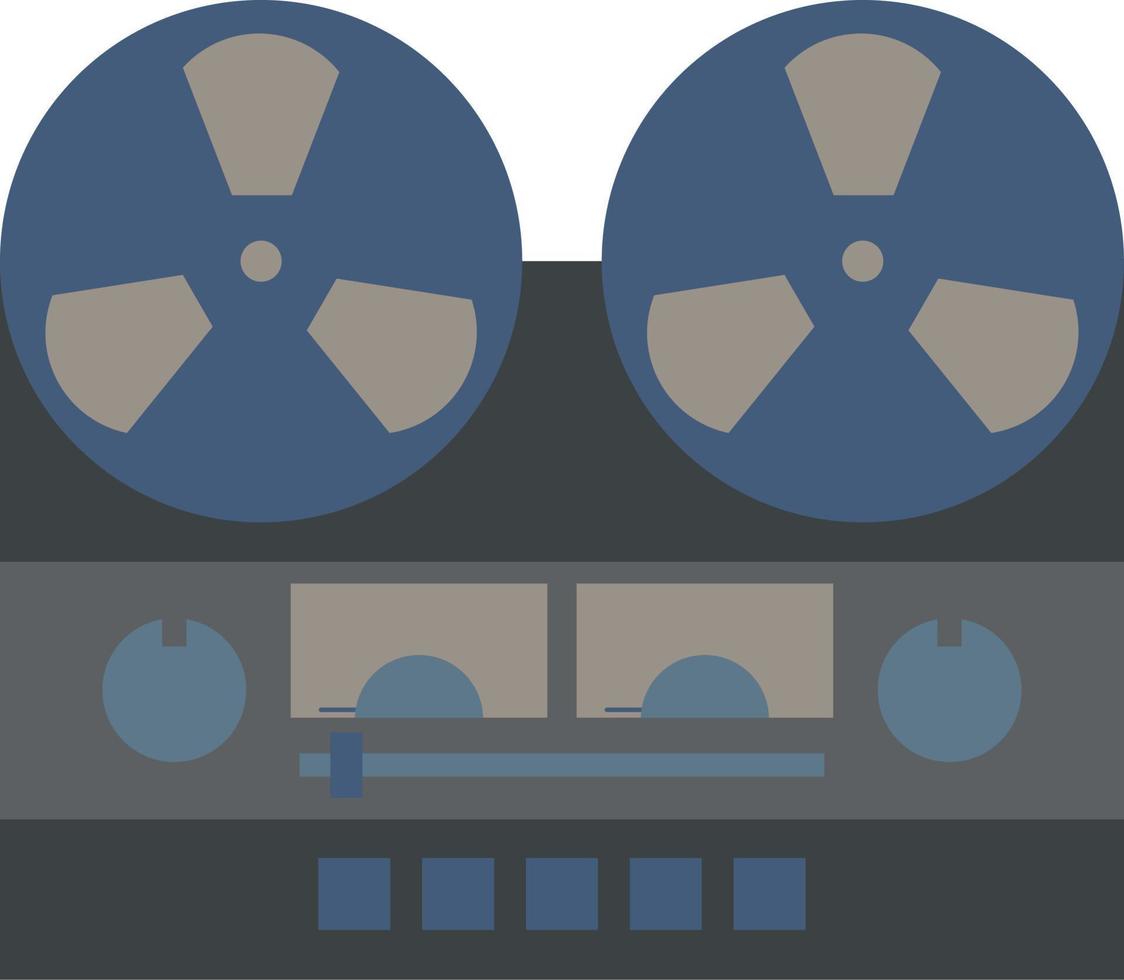The image is a detailed digital graphic depicting an animation-style old-fashioned movie projector, composed of geometric shapes. At the top, there are two reel-like circular objects reminiscent of film reels. These circles, primarily blue with beige central cutouts, contain three openings arranged symmetrically. Below the reels, the body of the projector features a combination of dark gray and lighter gray shades, segmented with blue squares and beige rectangles. Two light periwinkle blue knobs are situated at each end of the projector. In the center, there are two identical rectangular shapes, each with light blue semicircles. Additionally, beneath these, there is a horizontal adjustment slider, dark blue in color, suggesting controls for volume or light. Finally, at the bottom, five evenly spaced blue squares align horizontally across the dark gray base, adding to the intricate design features of this technological illustration.